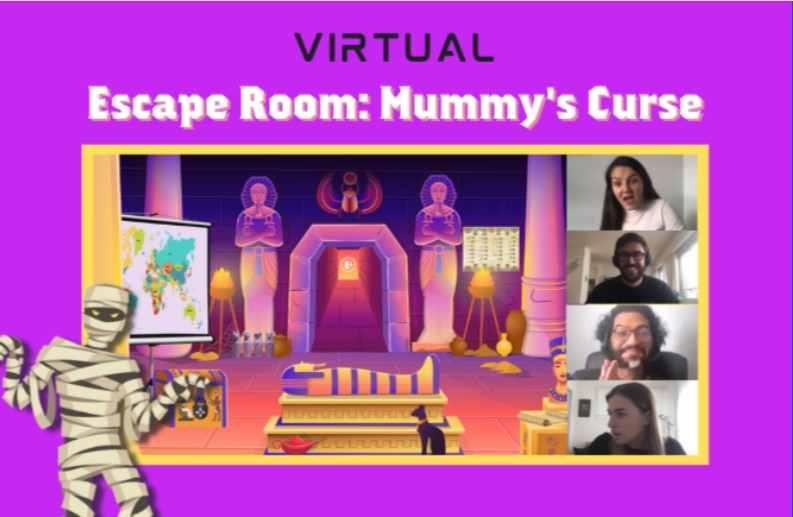The image captures a vibrant purple background with the word "VIRTUAL" prominently displayed at the top in black, capital letters. Directly below, in white letters, it reads "ESCAPE ROOM: MUMMY'S CURSE." Encased in a yellow border is a vivid digital scene reminiscent of a video game. At the forefront, a mummy lies on a table, surrounded by a dimly lit tomb with flickering lamps. Two mummy figures flank a doorway leading into a tunnel, hinting at an ancient Egyptian setting. To the bottom left of the central scene is a detailed cartoon depiction of a mummy with slanted yellow eyes and unwound bandages. On the right side of the image, four participants appear in a grid layout, reminiscent of a Zoom or Microsoft Teams call. They engage with the game; three face forward, with one woman glancing left. The participants include two men and two women, each against a plain white background, with the men notably wearing glasses.